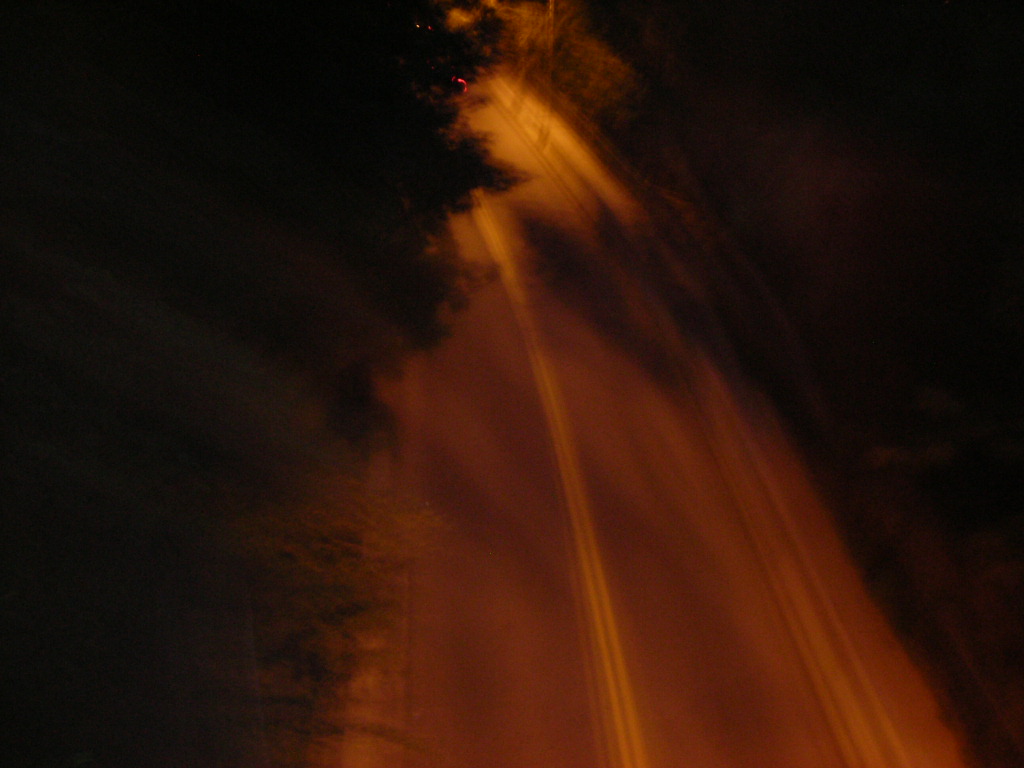The image is a color photograph taken at night, capturing a downward view of a road illuminated by streetlights from an elevated height, roughly equivalent to two stories. The vantage point suggests the photo could have been taken from a drone or a bridge, though the support structure is not visible.

The road stretches below, bathed in a yellow and orange tinge due to the nighttime lighting. A double yellow line runs down the center, creating a distinct separation between the two lanes of traffic. However, the lines exhibit a slight ghosting effect, likely caused by a slow exposure, with a faint second set of lines appearing close to the main ones, indicating camera movement during the long exposure.

On both sides of the road, dark masses of foliage—trees and bushes—crowd in, their outlines encroaching over the top of the road, casting shadows upon it. The right side of the road, as it curves to the left, features shadows from these trees, adding to the eerie atmosphere. There is a hint of red stoplights barely visible as a car rounds a corner, adding a dynamic element to the otherwise still scene. The interplay of the gold and yellow streetlight casts lighter and darker shadows across the road, enhancing the ethereal quality of the photograph.